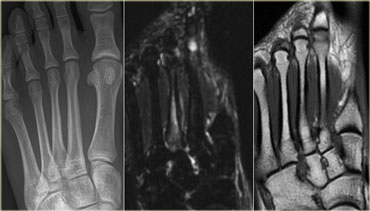This composite image features three x-rays of a foot placed side-by-side, each offering a distinct perspective and detail level. The leftmost x-ray displays a clear top view of the foot, including toes and part of the midfoot, with no immediately discernible breaks or damage. The bones are outlined in white with a gray interior. The center x-ray is notably darker, with bones appearing in black and gray, and it lacks the big toe, giving an impression of potential damage or absence. This middle image also has a white, blurry spot at the top, possibly indicating edema or swelling. The rightmost x-ray combines features of the other two: it has the gray bones with a darker outline similar to the center image, but also shows areas of the foot more clearly like the first one. Notably, the big toe is also missing in this image, and the bones appear thinner, hinting at possible severe trauma or previous surgical intervention. Overall, the collective images potentially suggest the progression or aftermath of a significant injury or condition affecting the foot.